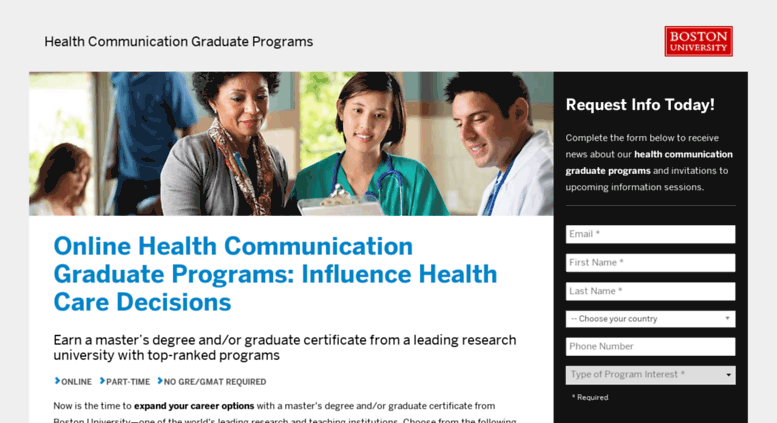This image features promotional content for Boston University’s health communication graduate programs. In the upper left corner, the title "Health Communication Graduate Programs" is prominently displayed. On the upper right, within a red box with white font, is the logo or name of Boston University. Below this, the image is divided into two vertical sections.

The left section includes an image and descriptive text. At the top, a photograph depicts three individuals examining a clipboard, emphasizing collaborative study or research. Underneath the main title, the text reads: “Online Health Communication Graduate Programs Influence Health Care Decisions,” highlighting the impact and online accessibility of the program.

The right section features a black box with the call-to-action text "Request Info Today." Below this, a statement prompts prospects to "Complete the form below to receive news about your health communication graduate programs," followed by six white input fields for potential students to fill in their details.

The overall design effectively combines visual elements and informative text to attract potential students to Boston University’s health communication graduate programs.